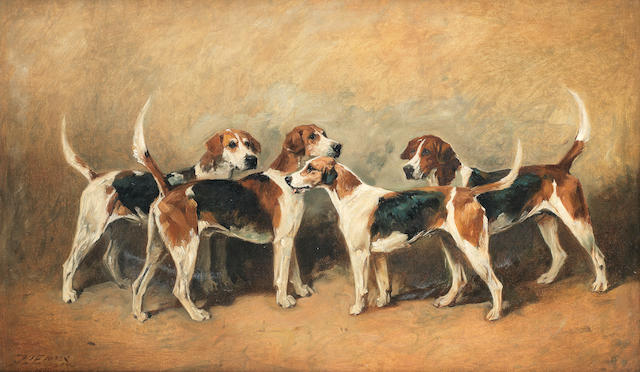The image depicts a richly detailed oil painting featuring four English foxhounds standing in an earthy, autumnal setting. The background is composed of warm tones of orange, yellow, and varying shades of brown, suggesting a natural, rustic scene with a brown wall and soil. All four dogs are positioned symmetrically, with two dogs on the left facing right and two on the right facing left, meeting in the center. The foxhounds have predominantly white bodies adorned with irregular patches of burnt orange and black markings. Each dog has distinct features: from one with a black ear to others with orange ears and white snouts. Their tails, tipped in white, are all up and wagging. One of the dogs appears taller than the rest, and another is slightly shorter, adding to the dynamic composition. The harmonious blend of tans, whites, and blacks on their coats, coupled with their alert postures and dropped ears, suggests they may be hunting dogs poised in a moment of attentive stillness.